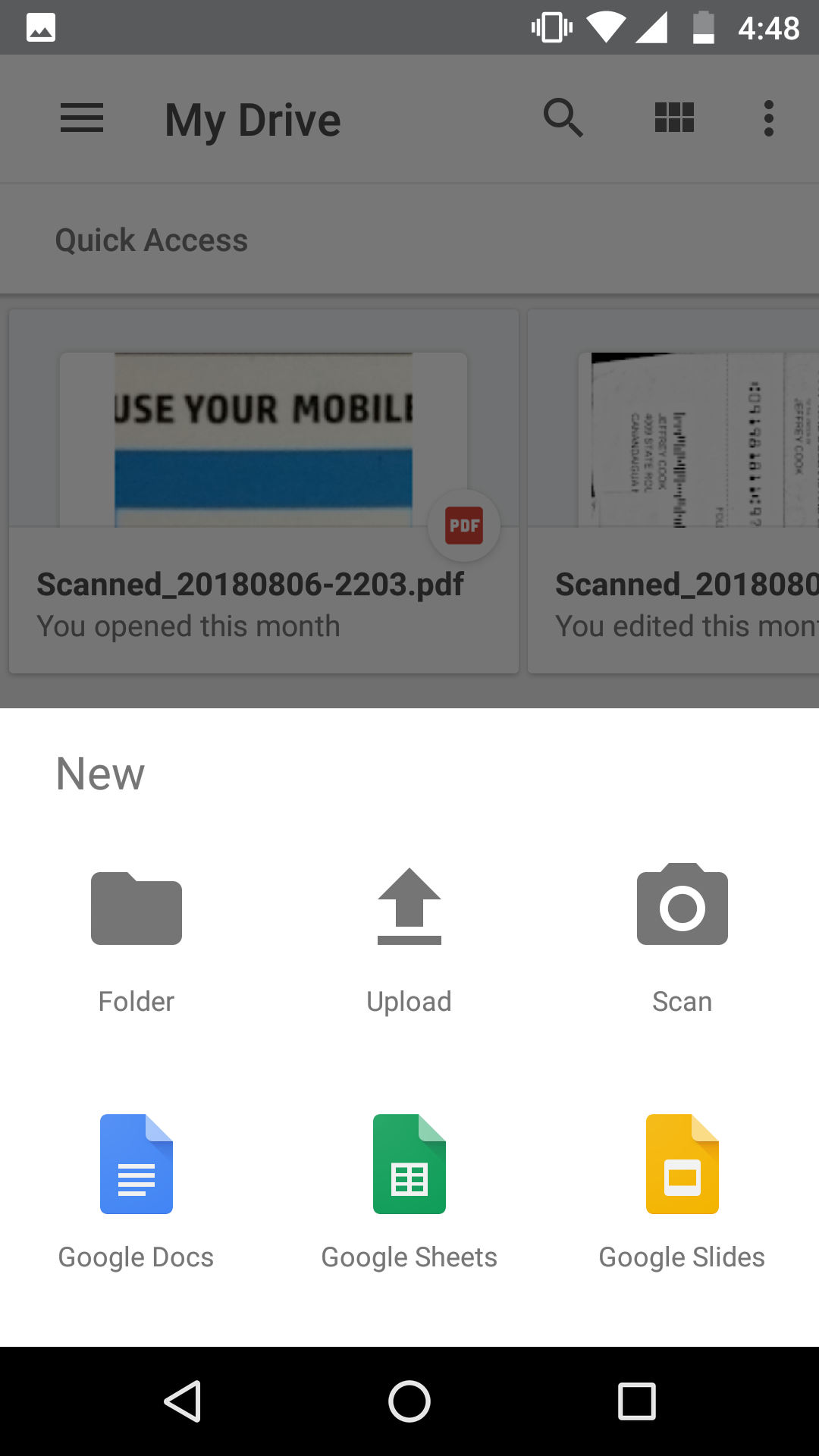This image depicts a smartphone screen showcasing Google Drive. 

The upper half of the screen features a translucent gray overlay. At the top of this section, a gray banner includes various icons. The first row reads "My Drive," accompanied by a magnifying glass icon for search functionality. Beneath that, the text "Quick Access" is displayed prominently in dark font. Below this, there is a blue rectangular button with the text "Use Your Mobile." Adjacent to that, on the bottom right, a white circle encloses an orange square with "PDF" inscribed in white font. Below this icon, a file name reads "scanned_20180806-2203.pdf," with a subtext in gray stating, "You opened this month." Another image and partial file name are visible to the right but are cut off midway. 

The lower half of the screen features a clean white background labeled "New" in gray font, followed by six icons arranged in two rows. The top row, in gray, includes icons for "Folder," "Upload," and "Scan," each represented by a folder, upward arrow, and camera icon, respectively. The bottom row displays colored icons for Google Docs (blue), Google Sheets (green), and Google Slides (orange). 

At the bottom of the screen, a black navigation bar is visible. It contains, from left to right, an arrow pointing left, a central white circle, and a white square on the right.